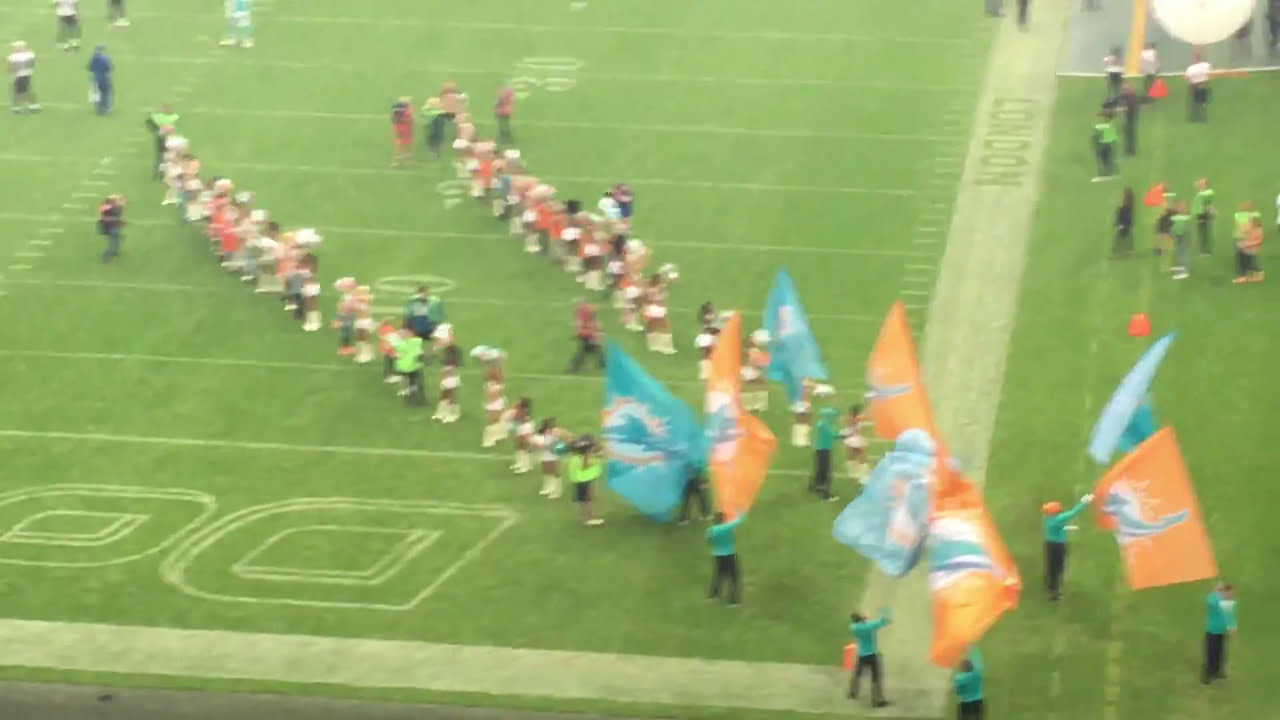This is a slightly out-of-focus photograph taken from a higher seat in the first bowl of a football stadium, capturing what appears to be a pregame event for the Miami Dolphins. The green football field is prominently featured, with two parallel lines of people forming a passageway diagonally from the bottom right-hand corner of the image towards about the 25-yard line. These individuals, possibly Miami Dolphins staff, are waving alternating orange and teal flags adorned with blue dolphins. Visible along the grass are the letters "D" and "O," likely spelling out "Dolphins," and the number "30" marking the 30-yard line. The word "London" is also visible on the field. The lower right corner features camera crew and event staff, while a bright light source can be seen in the upper right. The anticipation in the air suggests that players may soon enter for warm-ups.